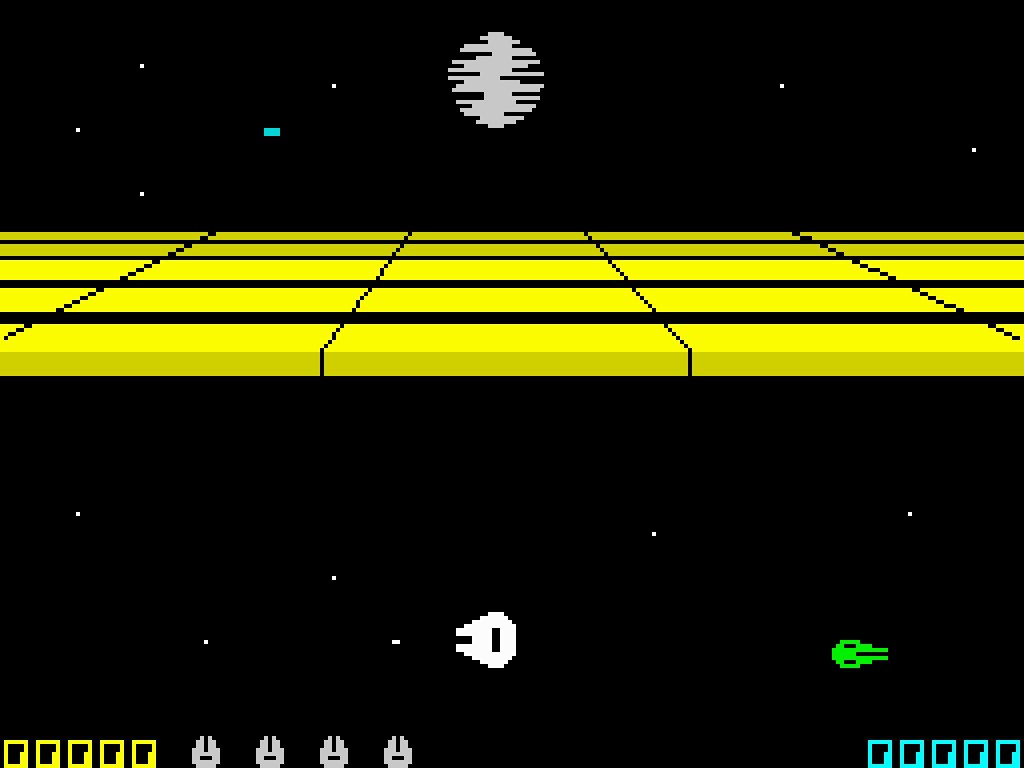This image appears to be a screenshot from an old arcade or video game, likely from the Atari era, and it may be a Star Wars-themed game. The background is entirely black, resembling the vastness of space, with scattered white pixelated dots representing stars. Dominating the upper middle of the image is a gray circular object with black lines extending inward, resembling the Death Star. Below this celestial body is a yellow grid-like plane laid flat, segmented into squares. 

Central to the gameplay visuals, beneath the yellow grid, are two spaceships: a larger white ship, possibly the Millennium Falcon, and a smaller light green spaceship to its right. At the very bottom of the screen, there are five yellow zeros in the left corner and five blue zeros in the right corner, which likely indicate score counters or lives remaining. This composition, coupled with iconic elements, suggests an immersive space battle scene.